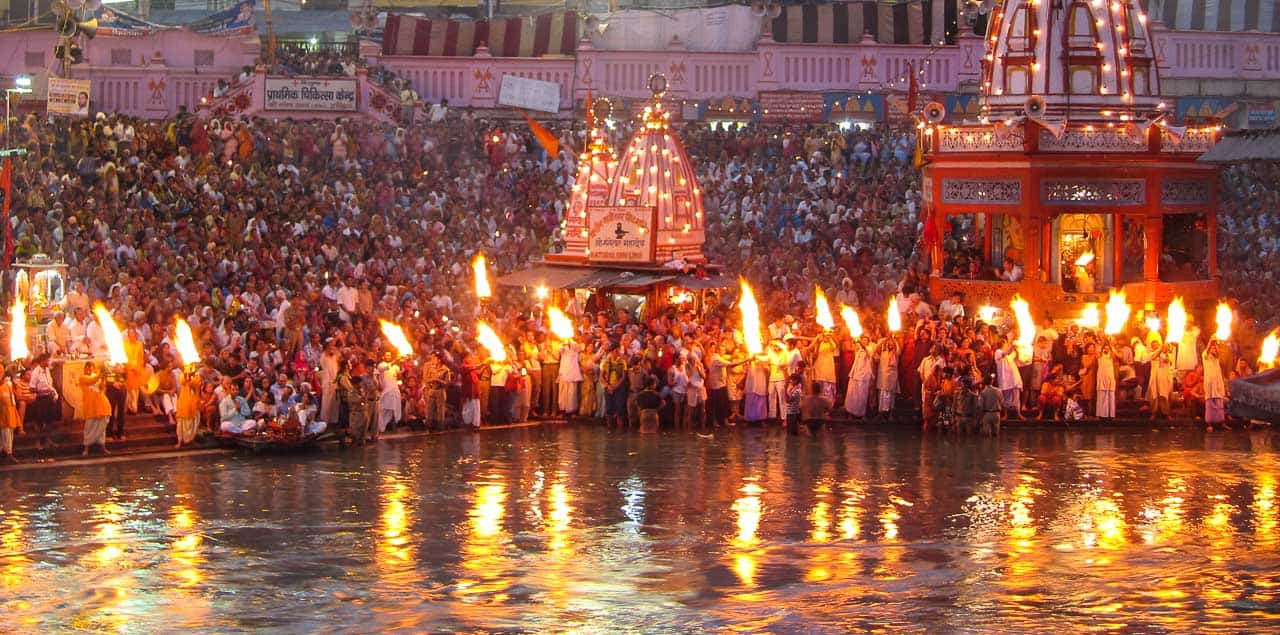This color photograph in landscape mode captures a vibrant evening festival or celebration, likely of Middle Eastern or Asian origin. In the foreground, there’s a man-made pond or fountain, its still surface beautifully reflecting the flames held by a dozen individuals along its edge. These individuals are adorned in traditional, billowy white garments, holding large open flame torches high on sticks. Behind them, a tiered arrangement of numerous spectators is visible, some sitting cross-legged with their hands together in a gesture of prayer. The air is filled with warm hues of reds and whites dominating the scene. In the background, a red, round gazebo with a white top is covered in shimmering string lights, adjacent to another structure resembling a small building crowned with a large dome, also adorned with festive lights. To the far side above the spectators, signs written in Arabic are posted on the walls, though their messages remain unreadable. Altogether, the scene is a mesmerizing blend of cultural elements, glowing lights, and communal gathering.